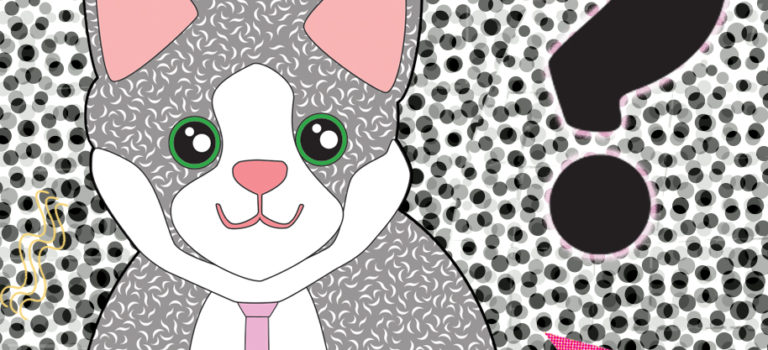The image is a simple, computer graphic-style illustration, almost cartoony and child-like, depicting a gray and white cat with green eyes. The feline’s ears display pink details, as well as its nose and mouth. A pink necktie or leash accessorizes the cat, resting against a white patch on its chest. The illustration emphasizes texture in the gray fur, providing a more detailed appearance. The cat is set against a black and white polka dot background, featuring a prominent question mark. The image is tightly cropped, showing only the top of the cat’s head, ears, face, and shoulders, with the ears being partially cut off. The cat seems to be smiling, exuding a playful and friendly demeanor.